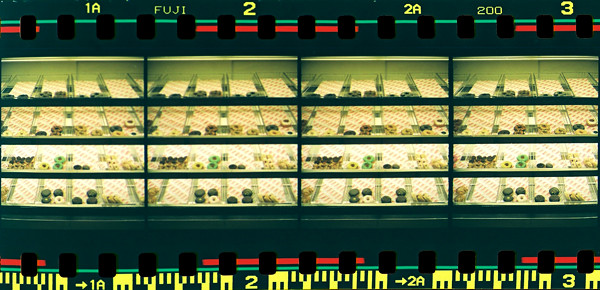This photograph captures a unique, vintage-style bakery display, reminiscent of an old Fujifilm negative slide. The image is divided into four identical sections, each showcasing a backlit glass cabinet filled with rows of donuts. The top and bottom borders of the photograph mimic the sprocket holes of film strips, with the top featuring 15 indentations and the text "Fujifilm" in yellow. Each section is labeled sequentially as 1A, 2, 2A, and 3. The cabinets are brightly illuminated, especially from the bottom shelves, displaying a variety of donuts in different colors including chocolate brown, white, green, and light tan for glazed. Some trays have more donuts than others, creating a dynamic visual of differing quantities. This detailed flow of repeated images evokes a sense of nostalgia, as if viewing a film negative of a cozy donut shop, possibly akin to a classic establishment like Dunkin' Donuts.